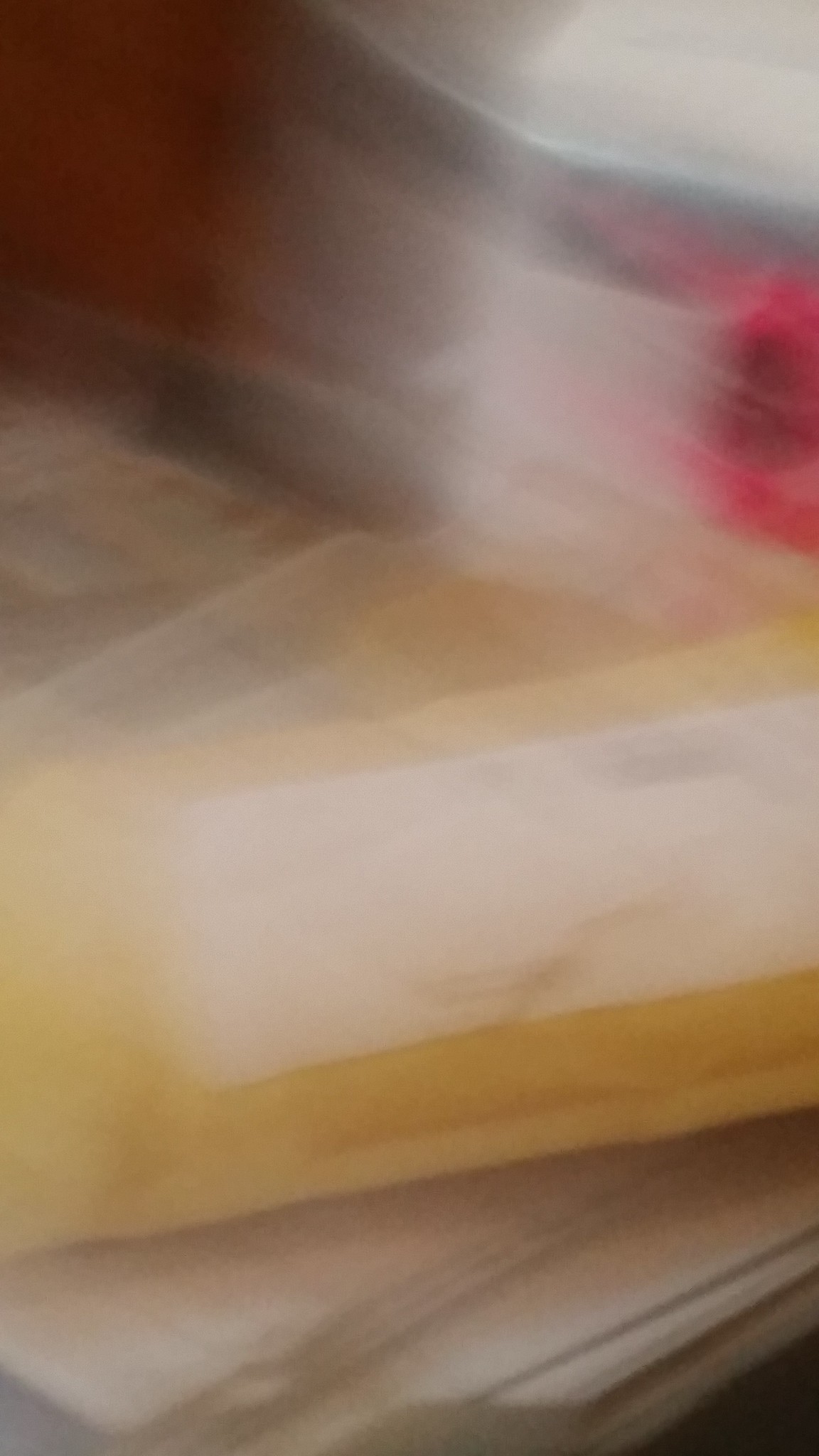The photograph is a highly blurry image, likely captured by someone in motion. It depicts a thick, almost cylindrical manila envelope with a prominent white label affixed to its surface. Although the image's blurriness obscures finer details, the envelope appears to be part of a larger pile of mail, evidenced by several other white pieces of paper visible underneath it. The background reveals various colors; the bottom right-hand corner features a very dark brown strip, while the top left adds a reddish hue. Additionally, the top right quadrant shows hints of pink and a white element. A faint whitish blur is present across the top edge of the photograph, further obscuring the scene.